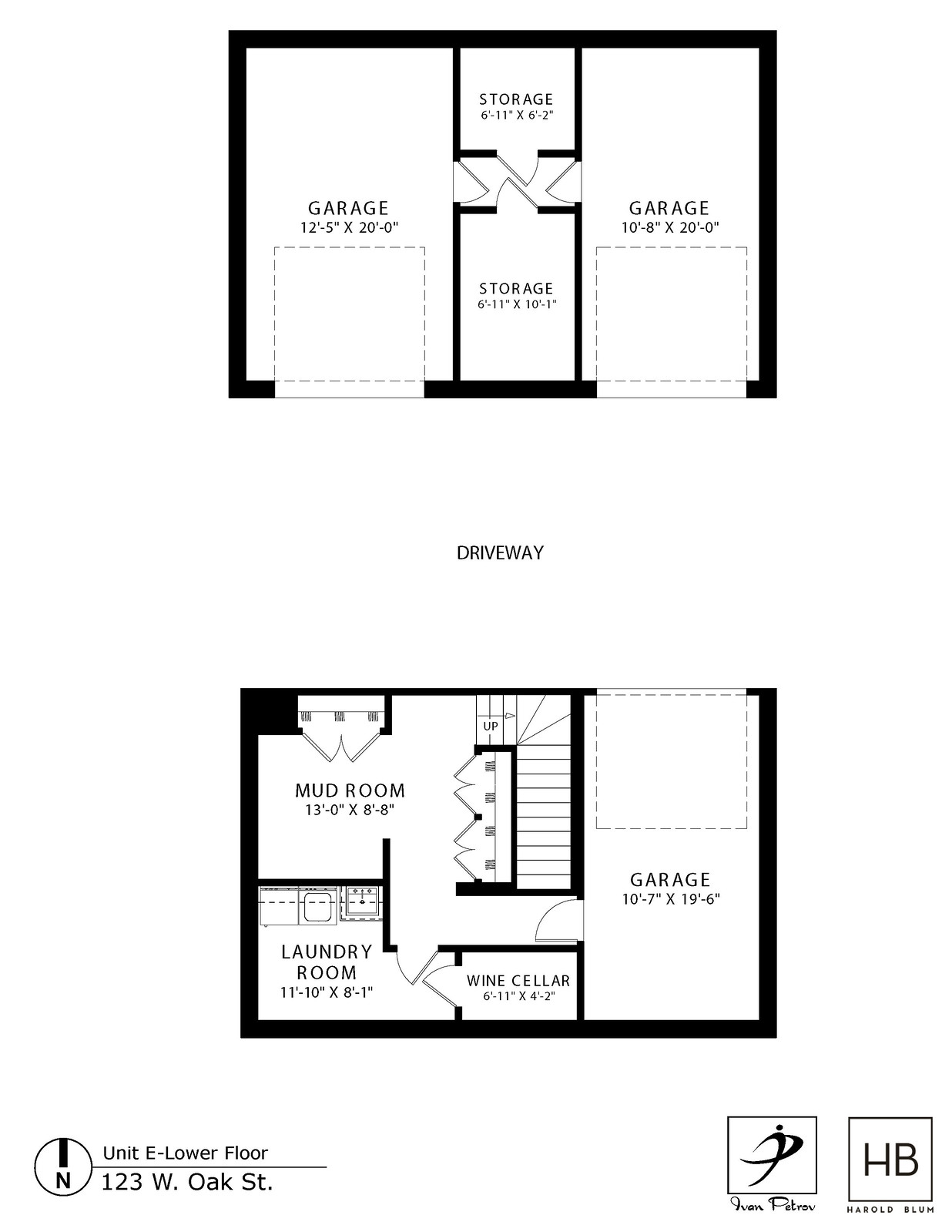This image captures the detailed layout of a residential unit labeled as "Unit E Lower Floor, 123 West Oak Street." The layout is depicted in two rectangular sections. The upper section shows a two-car garage, with labeled spaces "garage" on both the left and right sides. A dotted hash line indicates the pathway for cars to enter. Centrally located between these garages are two storage areas, with the top storage area being slightly smaller than the bottom one. Each garage is separated by walls, and access to the storage areas is provided by doors on each side of the garages.

The lower section of the image illustrates additional parts of the home. This includes another garage on the right side with an entry opening, and adjacent to this is a mud room on the left. The laundry room is situated in the lower left-hand corner of the layout. Additionally, a wine cellar is located within this section. The layout also showcases the placement of stairs and multiple closets, contributing to the home's functional storage and utility spaces. An emblem marked "Harbor" (abbreviated as HB) featuring a figure with a long arm wrapping around adds a distinctive branding touch to the floor plan.